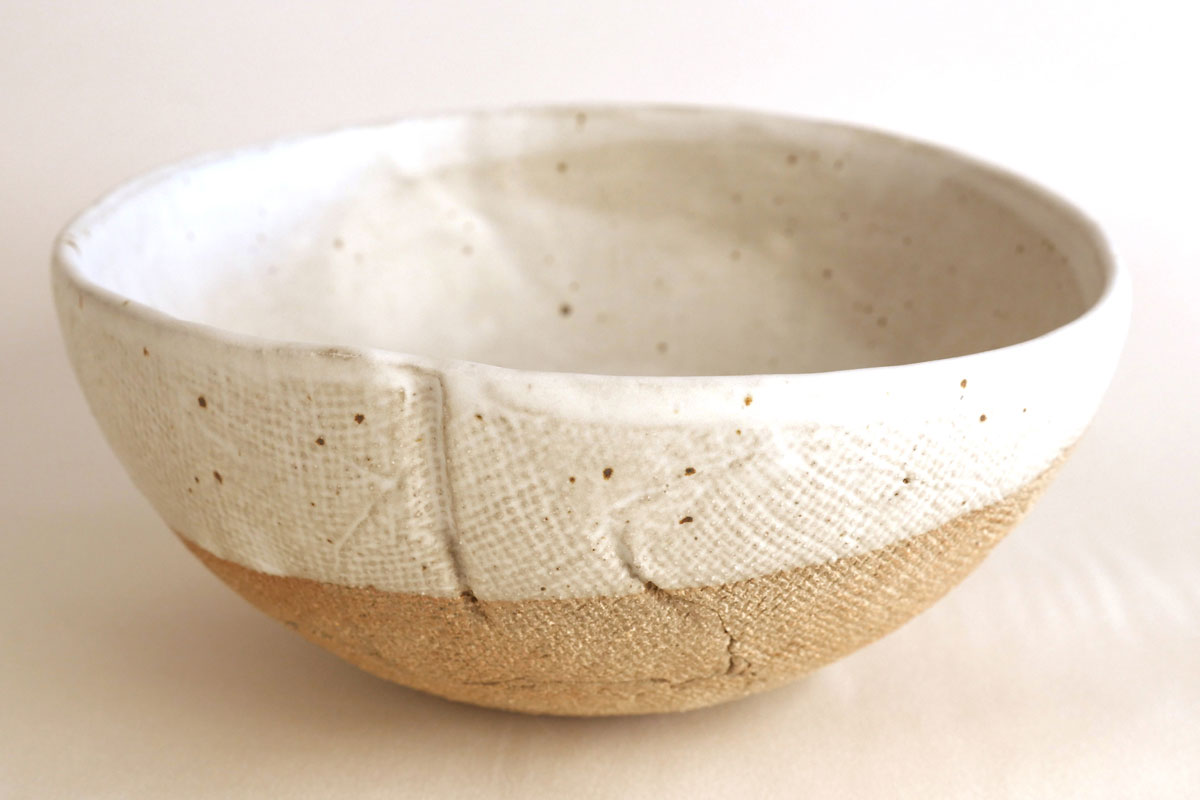In this photograph, a ceramic bowl takes center stage, positioned prominently on a light-colored wooden or cloth-covered table. The bowl, round and unfilled, showcases a two-tone design with a tan and white striped pattern encircling the upper rim. The body of the bowl transitions to a light brown hue, leading down to its cream-colored interior. Notably, the bowl appears to be well-preserved, despite a small crack and a few brown spots marking the white section. It sits alone in a minimalist, off-white setting, devoid of any utensils or food, suggesting its possible use for either decorative purposes or future culinary endeavors.